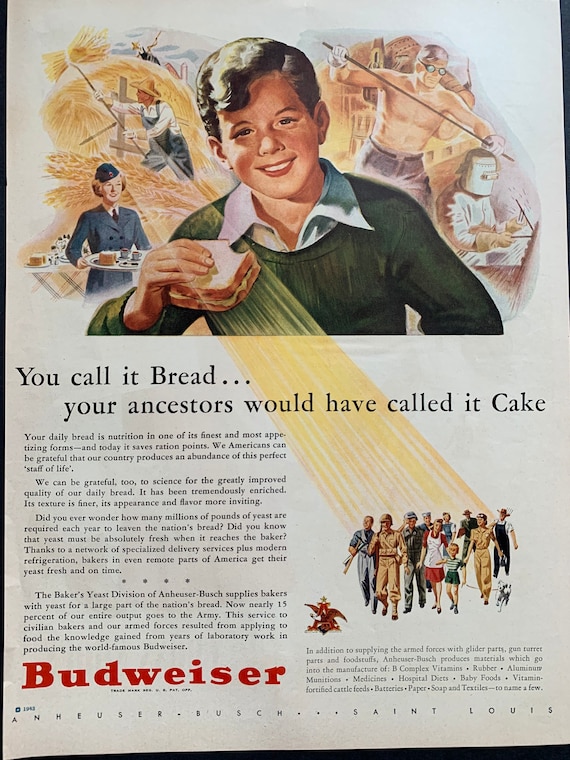This vintage Budweiser advertisement, possibly from the late 1950s or early 1960s, features a watercolor-style illustration with multiple scenes. At the top center, a young boy with dark hair, wearing a green sweater over a white collared shirt, smiles while holding a sandwich he's taken a bite from. Surrounding him are depictions of various American workers: a shirtless man working in a steel mill, a welder with a vintage helmet, a woman in a blue (possibly gray) uniform serving food, and a farmer bailing hay in a field. These images underscore the diversity and diligence of American workers.

In the upper-right section of the poster, the Anheuser-Busch logo with an eagle and an "A" stands prominently. Below these images, a bold statement reads, "You call it bread, your ancestors would have called it cake." Towards the bottom of the advertisement, a group of people from different walks of life look upward toward an array of sunlight, symbolizing hope and unity. The bottom left features the Budweiser name in red type, while the lower right corner contains additional information about the Baker's Yeast division of Anheuser-Busch. Scattered across the right and bottom, there are paragraphs of promotional text further emphasizing the American spirit and daily bread.